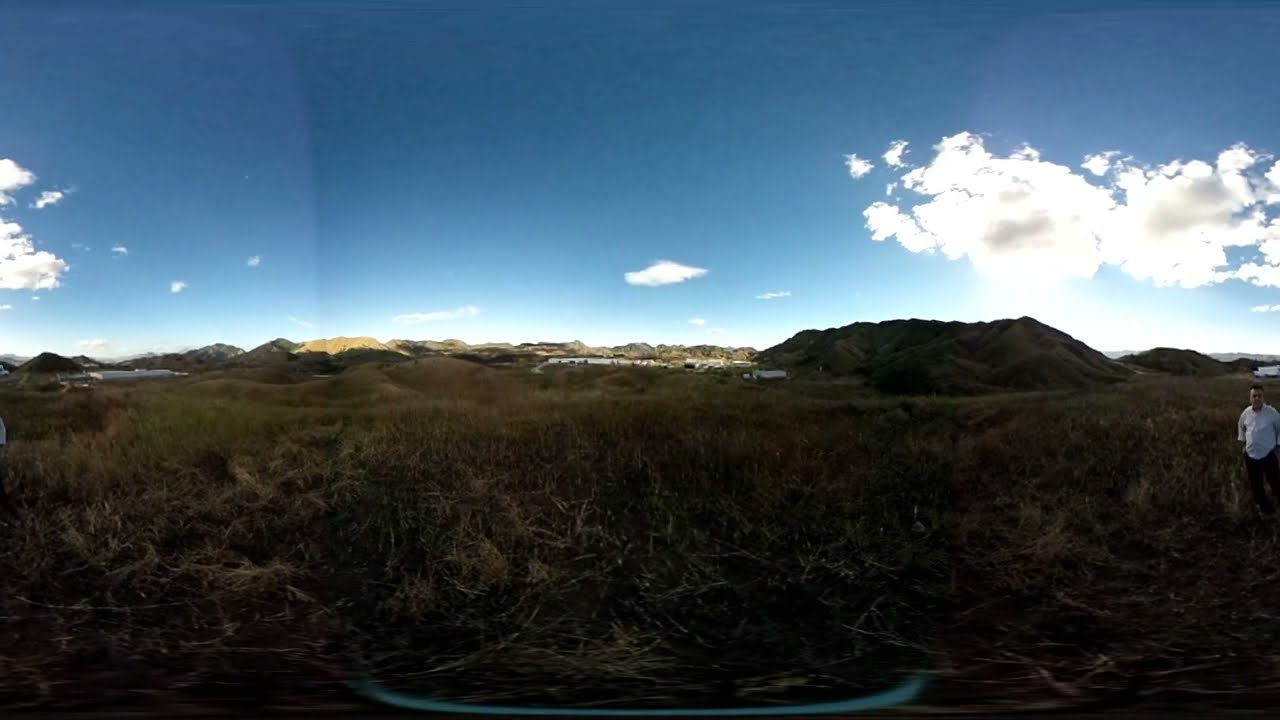The image showcases a vast, outdoor landscape with a panoramic view dominated by a medium blue sky adorned with a few clouds. The top half of the image captures this sky, where the sunlight peeks from behind distant foothills, hinting at a sunrise or sunset, and casting long shadows across the scene. Below, the terrain is mainly yellowish-brown, tallish grass, stretching widely and appearing wild and untamed, without any manicured lawns or trees. These rolling foothills might rise into mountains far in the background. The somewhat muted and dark quality of the image adds an atmospheric texture, though it's clearly sunny with the sun hidden by clouds to the top right. In the middle right portion of the photo, a figure stands out—a person wearing a white long-sleeve shirt and dark pants. The individual is partially in shadow, with their left foot forward and seemingly moving leftward while facing the camera. In the far distance, vague white structures are discernible, possibly sheds or a fence, though their exact nature is indeterminable due to the vastness of the view and the image's overall dark tone.